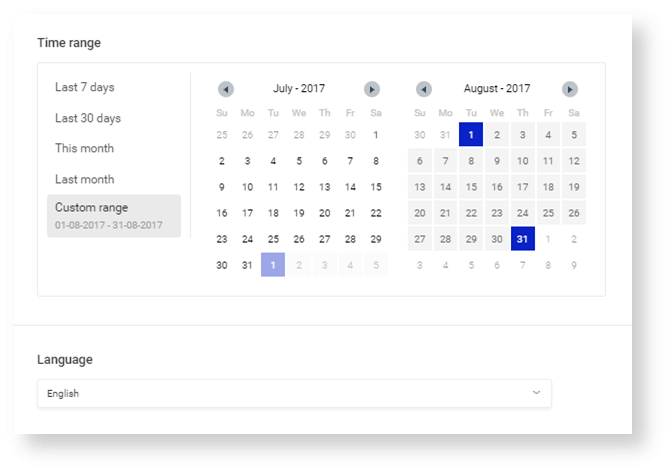The image depicts an interface with a predominantly white background, featuring a calendar function. On the upper left, the text "Time Range" is displayed in black letters. Below this heading are several selectable options in black text, organized vertically: "Last 7 days," "Last 30 days," "This month," and "Last month." At the bottom of this list, within a gray rectangle, is the option "Custom Range." Beneath this option, there is a date range displayed in faint gray letters: "01-08-2017 - 31-08-2017."

To the right of these options are two calendars, one for July 2017 on the left and another for August 2017 on the right. Each calendar header displays the month and year, flanked by two gray circles containing black triangular arrows, which presumably allow users to navigate between months. The days of the week are listed at the top in gray letters: S, U, M, T, W, T, F, S (Sunday through Saturday).

The calendar for July 2017 features black numbers denoting the days of the month, with the numbers of adjacent months faintly visible. The first day of August is faintly highlighted with a purple box. The August 2017 calendar similarly displays the days of the week and is entirely highlighted in gray squares, with the specific dates August 1 and August 31 highlighted in bluish squares with white text.

Below the calendars, separated by a thin gray line, is an option labeled "Language" in black letters on the lower left. Directly below this is a long, white rectangular box with the text "English" in black on the left side and a downward-facing arrow on the right, indicating the presence of a dropdown menu for selecting additional languages.